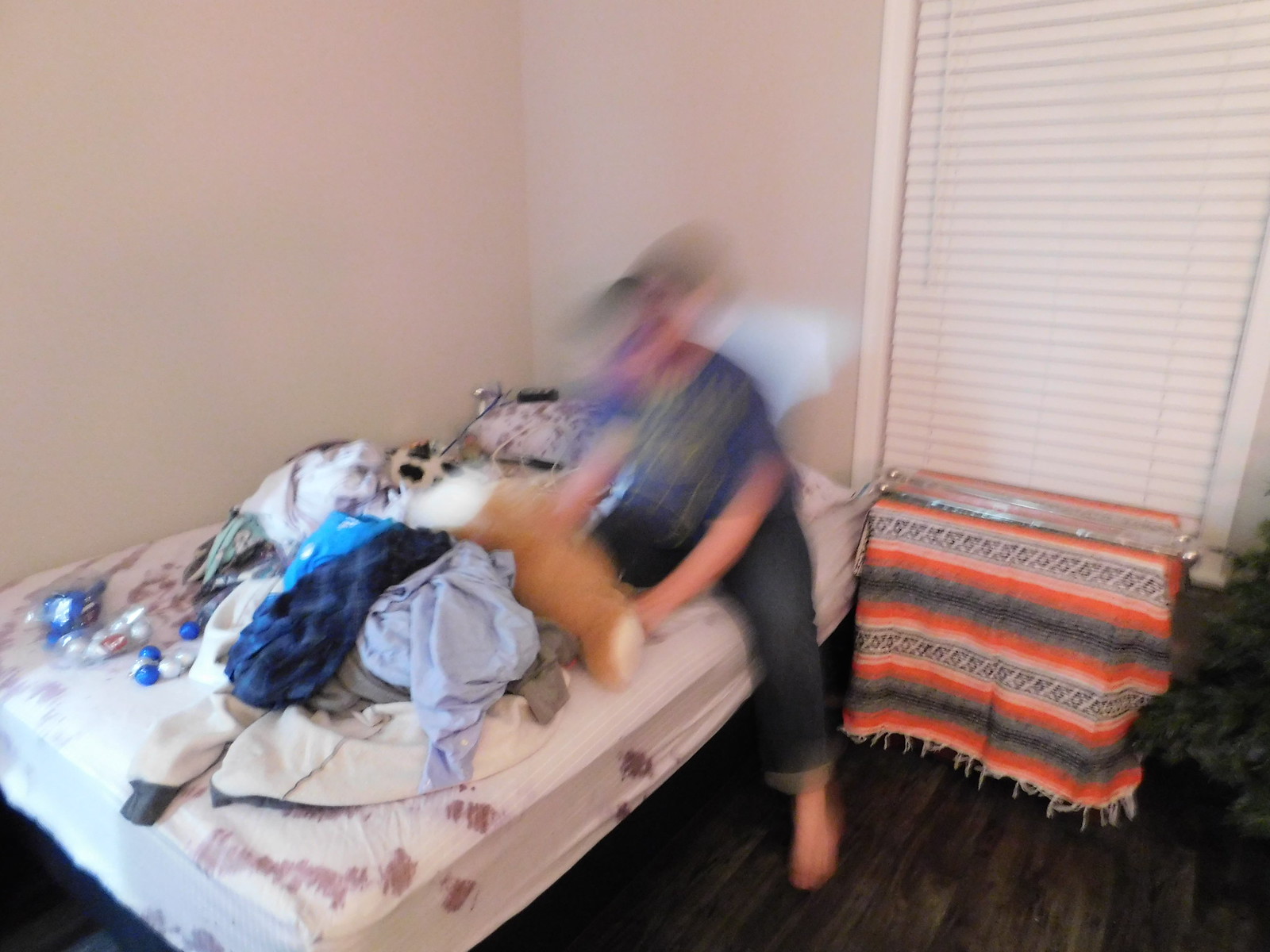In the blurry indoor photograph, a figure of a young to middle-aged woman is seated on an unmade bed overflowing with piles of scattered clothes. She is wearing a blue t-shirt with yellow text, cuffed jeans, and no shoes, exposing her feet on the wooden floor. The woman's face and head are particularly blurry, suggesting movement. The room has beige, possibly peach-colored walls and wooden flooring. To her right, a large, closed window with white horizontal blinds occupies much of the wall. Draped over a nightstand near the window is a colorful, Mexican-style Serape rug in shades of orange, white, gray, and black. The bed, covering much of the lower-left corner of the image, is cluttered with various blue garments and other items, including a couple of water bottles, emphasizing the disarray of the setting.